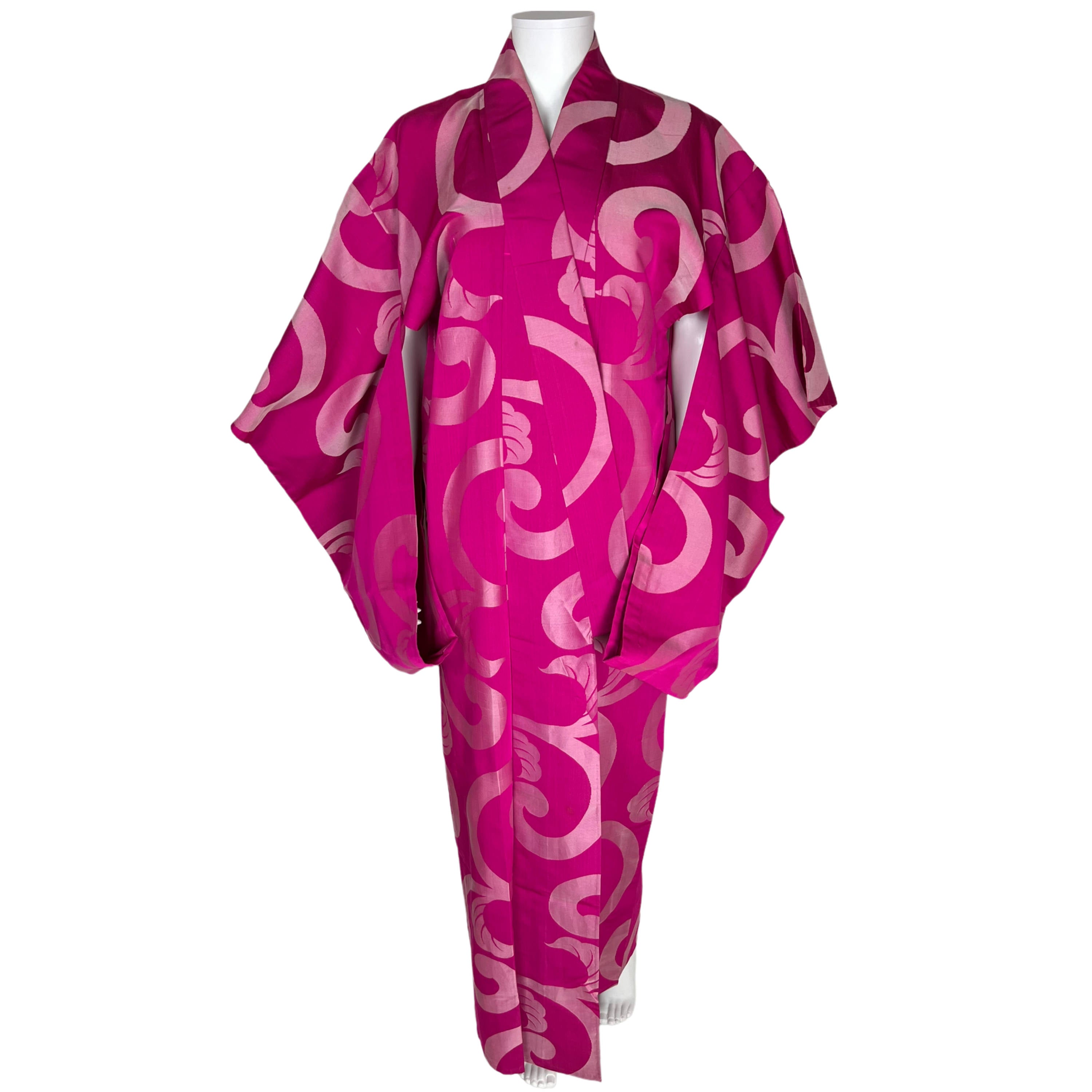The image features a traditional kimono, a robe-like garment that extends down to the ankles. The kimono is dark pink with various light pink semi-circle designs and lacks a sash, hanging freely with its right side folding over the left. Its long, flowing sleeves create a dramatic effect. The garment is displayed on a white mannequin, which has visibly articulated arms and legs but no head. The background is a flat white, giving the impression that the kimono is floating in an empty void, a common technique for online commercial listings.